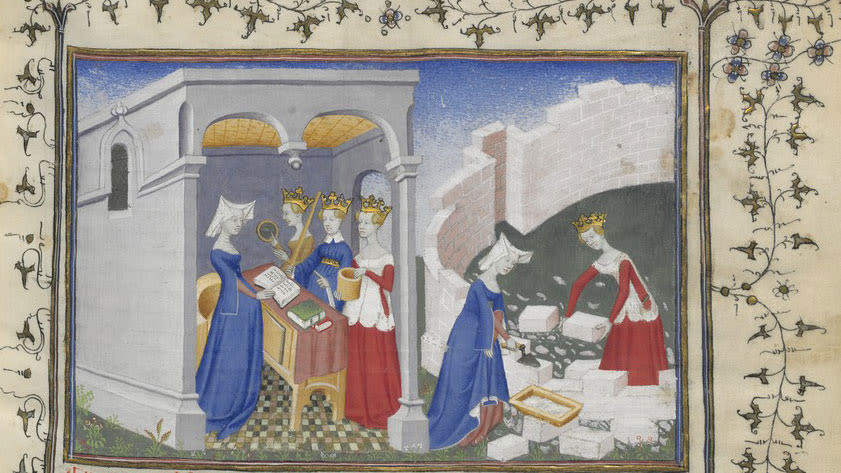The medieval-style painting, set on a tan wall adorned with flowery banners and vine motifs with darkish gold leaves, is encased in a decorative dark gold frame. The painting is rectangular and horizontally oriented, slightly skewed to the left. It depicts two distinct scenes with a group of women.

On the left, within a room, a woman in a blue robe dress, and white headpiece stands behind a table with an open book. Before her are three women: one in a red dress holding a bucket, another in a blue dress holding a stick, and the third, further back, in a gold dress holding a mirror.

On the right, outside, is a Colosseum-like structure where a woman in a red and white dress, adorned with a crown, is placing bricks on the wall. She is assisted by another woman in a blue dress with a white headpiece, who appears to be applying cement. The background includes a blue sky, suggesting an outdoor scene.